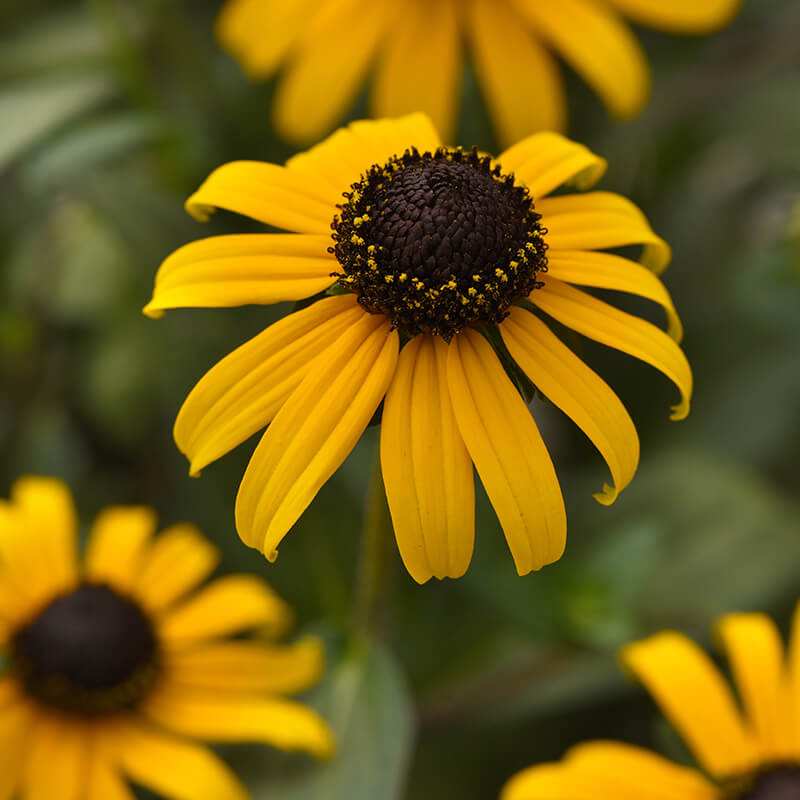This is a detailed close-up photograph of a single sunflower. The focal point of the image is the sunflower whose yellow petals are downturned and slightly curled under. The flower's center features a deep brown eye ringed with small, yellow inflorescences that add to its detailed texture. The petals, reminiscent of those found on daisies, fold away from the head of the flower, showcasing both their smooth appearance and subtle linear markings. The composition suggests a natural setting with a blurred background filled with green foliage and stems, punctuated by the vague, blurred outlines of three additional sunflower blooms situated in the upper middle, lower right, and lower left parts of the image. The background, with its brown and green hues, complements the vibrant, detailed centerpiece, adding to the serene and lifelike quality of the photograph.